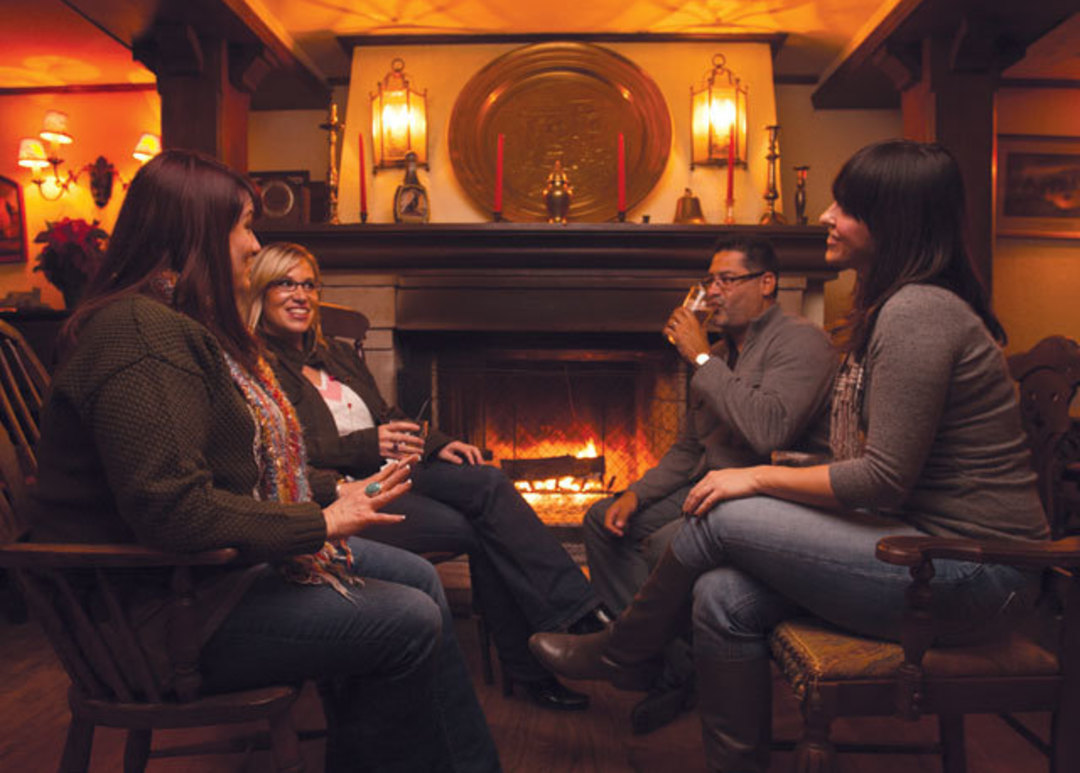In this warm and inviting scene, four people—three women and one man—are gathered around a fireplace, deeply engaged in conversation. The group is seated in a square-like arrangement with two people on the right and two on the left. On the right, a man with short black hair, black glasses, and a gray top is sipping from a transparent glass, possibly a beer, while sitting on a cushioned old-style wooden bench. Next to him is a woman wearing black leather boots, blue jeans, a gray top, and a scarf, sitting with her hand on her lap.

On the left side of the image, two women are seated in wooden chairs. One woman, dressed in a multicolored scarf and a green shawl-like jacket over blue denim jeans, sits closest to the camera. Behind her, another woman with blonde hair, black glasses, and a white top, who is wearing slacks, is captured smiling. The room emanates warmth from the lit fireplace in the background, which is framed by a large wooden mantel adorned with red candles, diffused lanterns, and a decorative figurine. The entire setting is bathed in a cozy glow from numerous warm-colored lights, accentuating the wooden theme that envelops the space. The attire of the people, featuring jeans, boots, and scarves, along with the modern yet rustic decor, suggests that the image is set in a contemporary, yet nostalgically-inspired room.